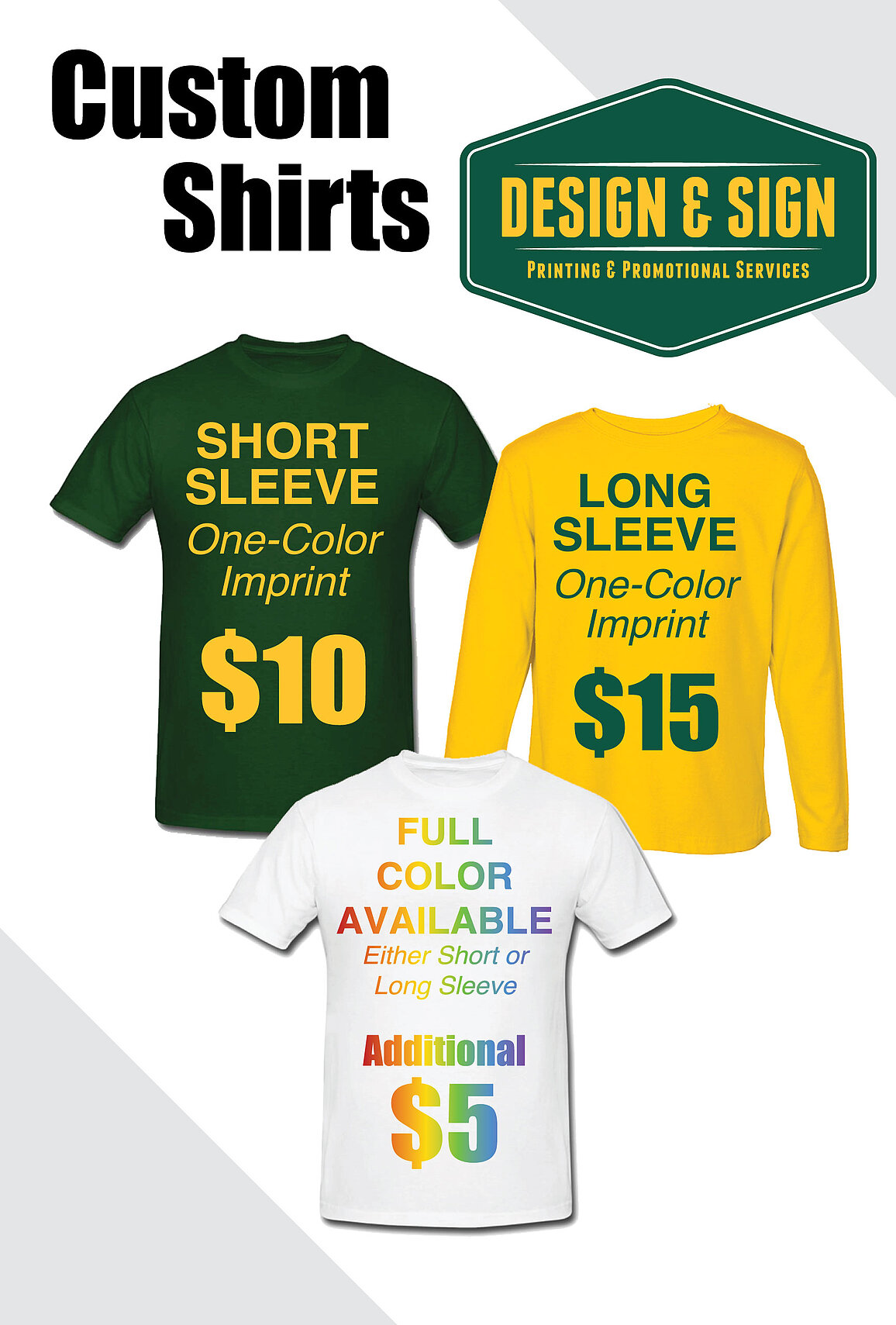This advertisement showcases custom shirts from "Design and Sign, Printing and Promotional Services." It features three distinct shirt options: a green short-sleeve crew neck with a one-color imprint priced at $10, a yellow long-sleeve crew neck with a one-color imprint for $15, and a white short-sleeve crew neck offering full-color printing for an additional $5, available for both short and long sleeves. The ad is framed with gray triangles in the corners, enhancing the visual presentation and emphasizing the detailed pricing and service information.